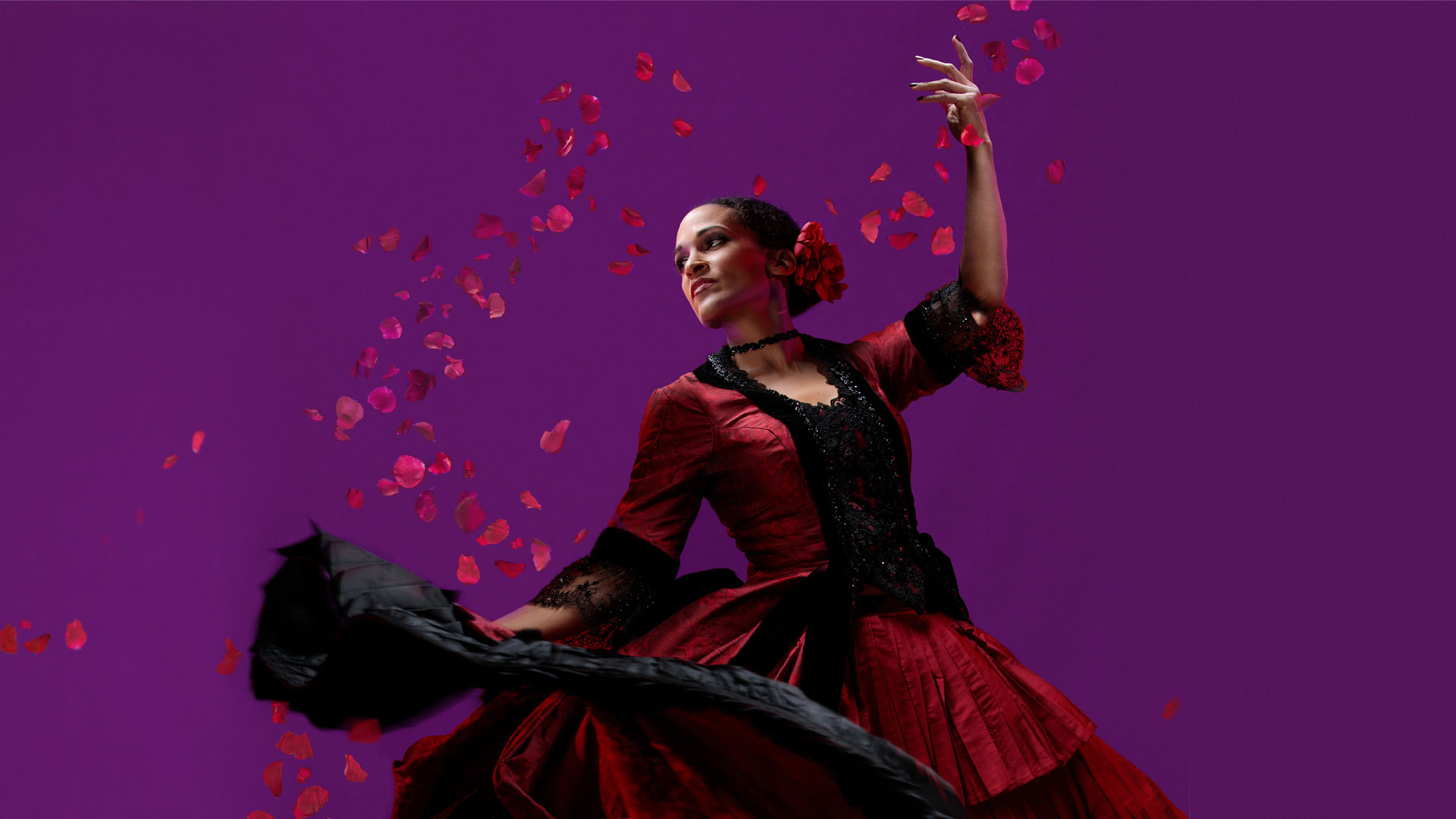In this captivating image, a Spanish flamenco dancer takes center stage against a light purple backdrop, creating a vivid contrast with her striking attire. The dancer, adorned in a stunning red dress with a black lace bodice and a flared skirt, skillfully holds out the bottom of her dress with her right hand, revealing its intricate black underside. Her left hand is raised gracefully in the air, heightening the classic flamenco pose. She has black hair styled in a bun, embellished with red flowers, which complement the vibrant rose petals scattered around her, suggesting a dynamic motion as if the petals were recently thrown. Her intense gaze is directed to her left, focused on something in the distance, adding an element of mystery and allure to the scene. The image is artistically framed with the dancer perfectly centered, making the bold colors of red, black, and purple pop brilliantly, creating a mesmerizing visual composition.